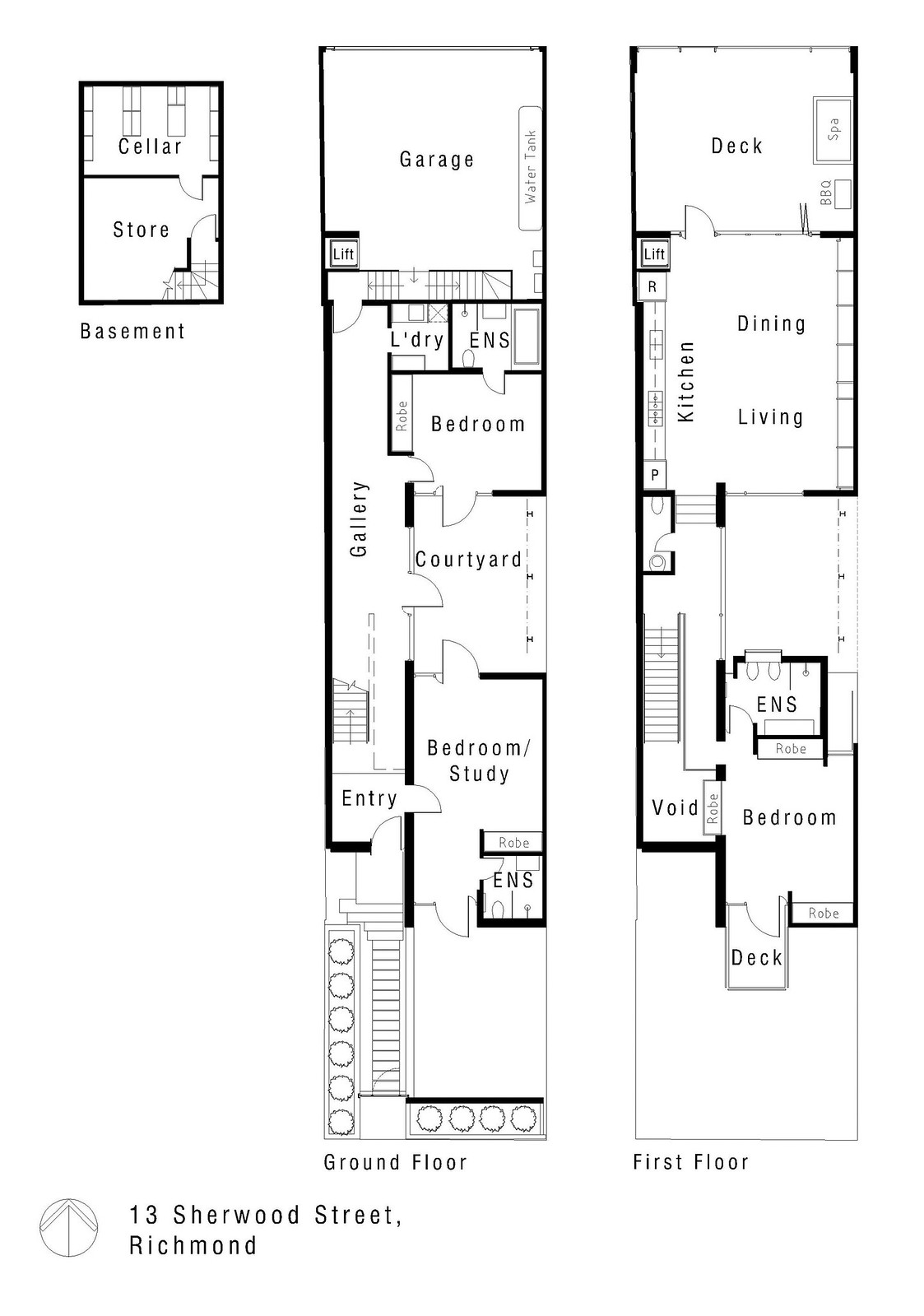This detailed architectural blueprint illustrates a two-story, long, narrow house with a front-facing garage. The basement, which appears to be potentially located beneath the garage, comprises a cellar and a storage area, accessible via a small, curved stairwell along the outer wall, likely starting from the garage. The ground floor features an entryway leading to a laundry room, followed by a long hallway. Adjacent to this hallway is a bedroom, and a courtyard is situated beside a versatile room labeled as a bedroom/study. The upper floor boasts a deck positioned above the garage, alongside the main living spaces, including a kitchen, dining room, living room, and an additional bedroom. This design emphasizes vertical living, with the kitchen and primary living areas strategically placed on the upper level.